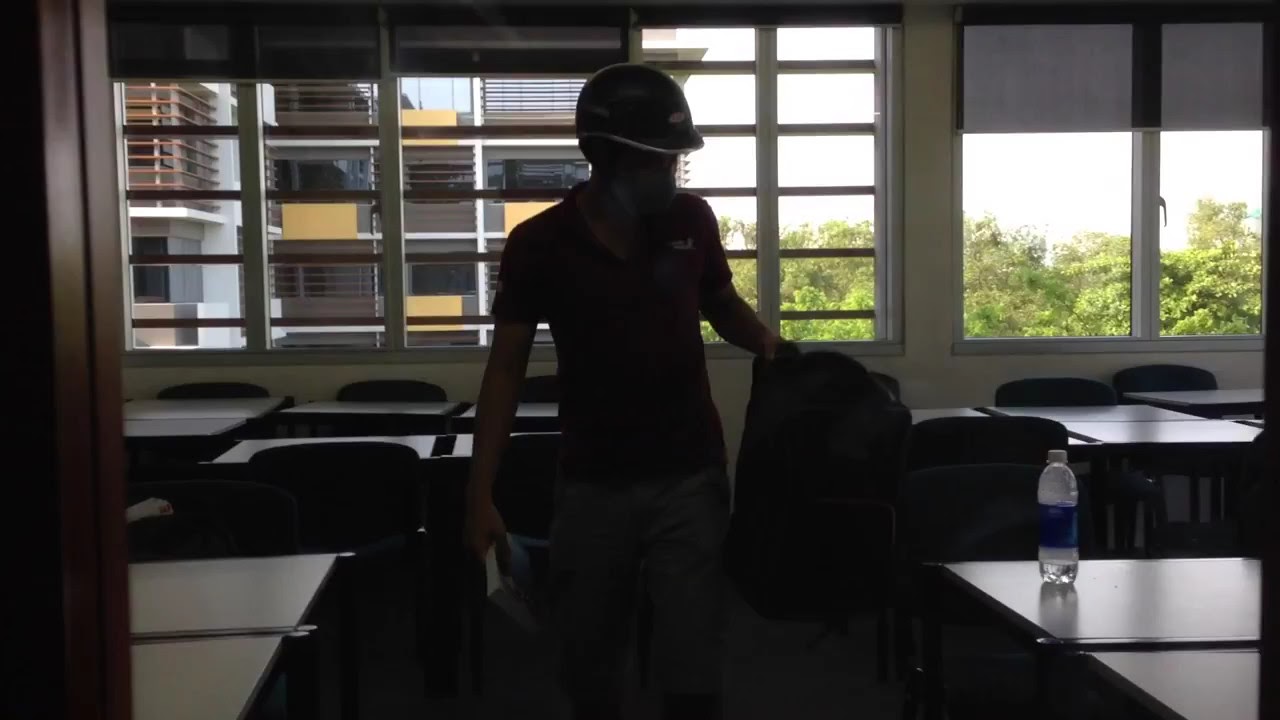The image depicts a young white male, likely a student, standing in a dimly-lit room that appears to be a classroom or an office. He is directly in the center of the image, adorned with a black hard hat featuring a white line on the bill and wearing a mask that resembles an N95. His attire includes a red short-sleeved polo shirt with some writing on it and neutral-colored shorts. In his left hand, he holds a black backpack, which he's holding somewhat away from his body, and in his right hand, he carries a paperback book.

The room is filled with numerous square student desks with accompanying pull-out chairs, all of which are unoccupied. The floor is carpeted, and there is a notable absence of artificial lighting, contributing to the room's overall dark ambiance. To his right on one of the desks, there is a plastic water bottle with a blue label and a white top.

In the background, the room features large windows that reveal two distinct views: to the left (from the viewer's perspective), there is a white building with black windows and balconies equipped with metal bars and yellow squares. To the right, there is green leafy vegetation, including trees and bushes. The windows directly behind the man have horizontal metal bars across them and vertical slats, indicating the bars are on the building's exterior. The top third of some of these windows is covered by shades, and the daylight streaming in emphasizes the contrast with the room's darkness.